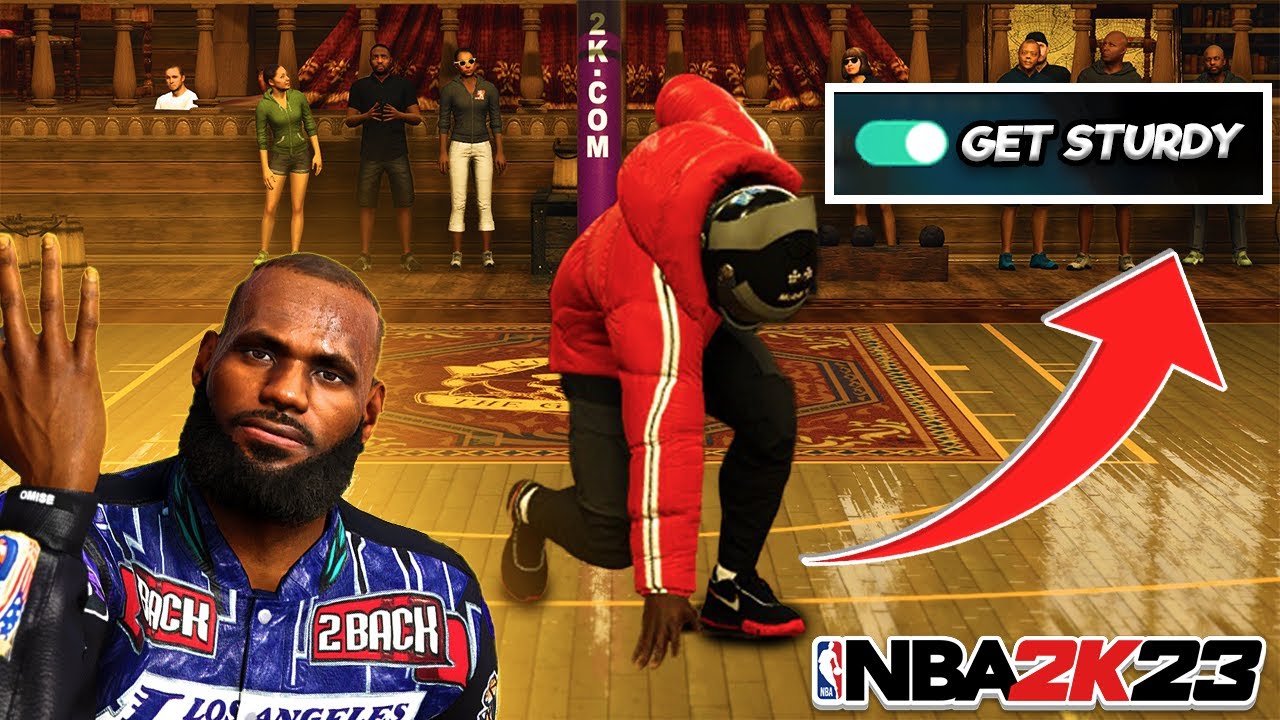In this vibrant and dynamic image from a video game, the background features a wooden floor partially covered by a predominantly red rug. Just beyond the rug, a wooden platform supports a group of people - three on the left side and five on the right. Centered on the platform is a purple vertical banner adorned with white text that reads "2k.com" from top to bottom. The setting is enclosed by ornately carved wooden banisters atop a wooden wall, with one individual in a white shirt visible on the far left side.

At the forefront of the image, a man is striking a dynamic pose. He is dressed in tight black pants paired with black shoes that have distinct red bottoms and a large puffy red jacket featuring a white and black stripe down the sleeve. A black helmet completes his ensemble. His left knee is bent with his foot flat on the ground, while his right knee is bent with only his toes touching the floor. Leaning forward, he supports himself with his right hand on the ground, while his left arm extends behind him.

Dominating the center of the frame is a red arrow with a white outline, curving upward to the right, pointing towards an overlay with a dark blue and black gradient background and a white outline. This overlay contains a teal blue pill-shaped selection button with a white circle on the right. To the right of this button, bold 3D black shadowed white text in all caps reads "GET STURDY." Additionally, there are two overlays of people positioned at the bottom corners of the image - one in the bottom right and the other in the bottom left, completing the detailed scene.